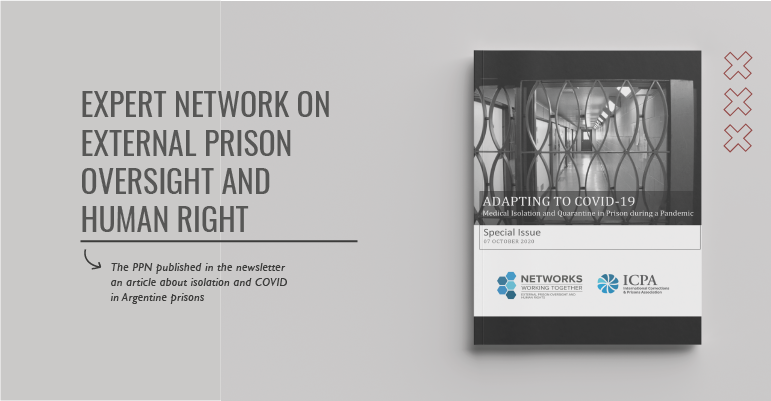**Caption:**
This image appears to be either an advertisement or a website header, set against a gray background and framed in a rectangular format. 

On the left side, aligned to the left and presented in large, uppercase black letters, the text reads:

- "EXPERT NETWORK ON"
- "EXTERNAL PRISON"
- "OVERSIGHT IN"
- "HUMAN RIGHT"

Beneath "HUMAN RIGHT," a hand-drawn black line with an arrowhead curves downward, leading to a paragraph in smaller, left-aligned black lettering: "The PPM published in the newsletter an article about isolation and COVID in Argentine prisons."

On the right side of the image, there is a photograph of a window embedded in a prison door. The window features uniquely shaped oval bars and seems to offer a view down a pristine and glossy corridor of what is presumably a prison, characterized by its industrial appearance and tiled surfaces.

Below the window, the white text reads: "Adapting to COVID-19, Medical Isolation and Quarantine in Prison During a Pandemic, Special Issue."

At the bottom left corner, the word "Networks" appears; at the bottom right, "ICPA" is displayed. There is additional writing beneath these words, but it is too small to be legible.